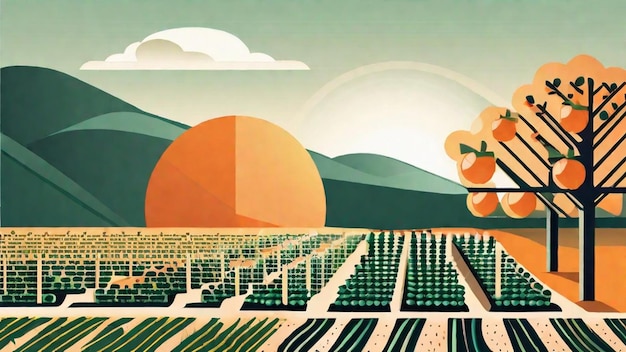This digital, stylized image depicts a surreal garden or farm landscape with an emphasis on geometric forms and abstract representations. On the right side, there are trees with unusually straight trunks and branches that extend only at precise 90 and 45-degree angles. These trees bear enormous orange fruits that dwarf even the size of pumpkins. The ground is tan, bisected by rows of plants made from green circles and lines, the purpose of which is left to interpretation. Rising from this tan soil are thin, tan lines that likely represent wooden posts. To the left, the rows of plants appear lighter green, while on the right, they are a darker green. In the background, undulating green hills are set against a sky with a gradient of green hues and a significant light effect just off-center. Dominating the scene is a colossal orange circle hovering over the field but in front of the hills, disjointed from the traditional sun, adding to the enigmatic atmosphere of the image. Above, a faint, light gray rainbow arcs across the sky, coupled with a large white cloud, contributing to the otherworldly feel of the scene.